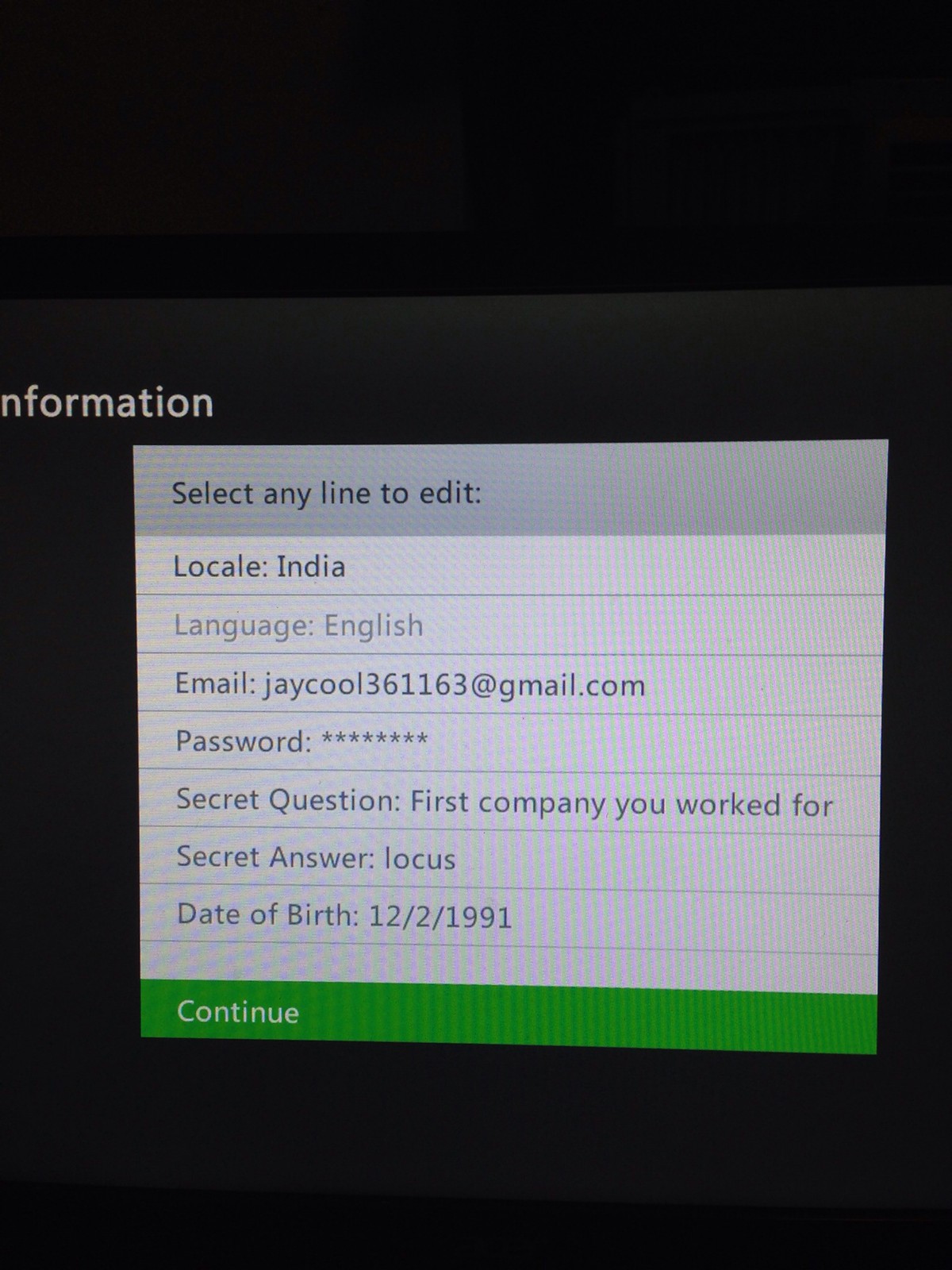The image is a vertical screenshot of a computer screen with a black background. At the center, there's a rectangular box. The top part of the box has a gray bar labeled "Select any line to edit." Below the gray bar, there are several white bars with different labels and corresponding information. The first white bar says "Locale: India." The next white bar reads "Language: English." Following this, there's another white bar with the email "jcool361163@gmail.com." The next white bar displays the "Password" hidden with asterisks. The following white bar contains the "Secret Question," which reads "What was the first company you worked for?" and the "Secret Answer," which is "locus." The last white bar lists the "Date of Birth" as "12-2-1991." At the bottom of the box, there is a green bar with the text "Continue."